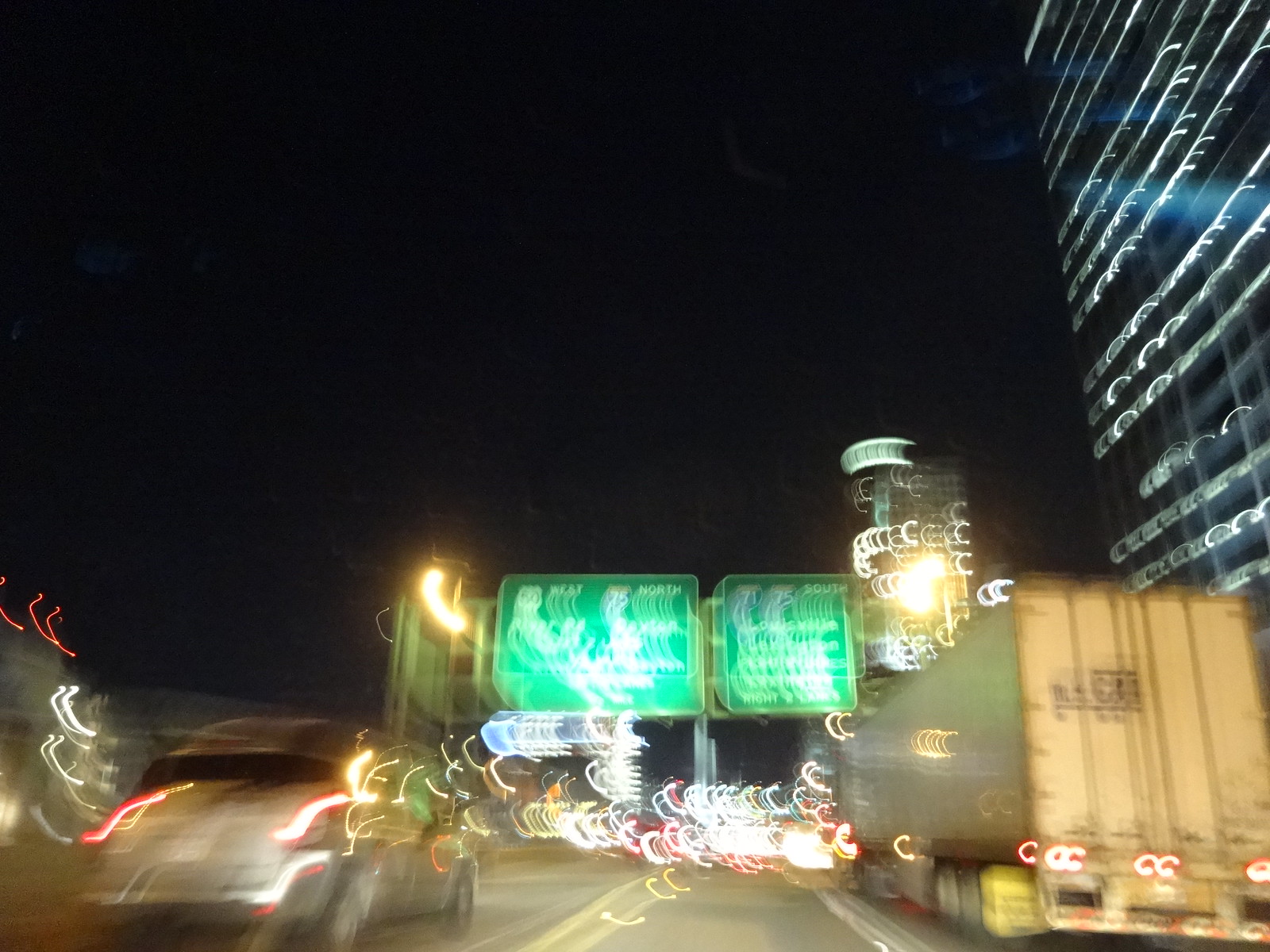Captured from what is likely a dashboard camera, this blurry nighttime street scene shows a bustling urban environment. The pitch-black sky envelopes the scene, with the sole source of light being a large, illuminated building on the right side of the image, possibly a high-rise or apartment complex. The photo, possibly taken while in motion, reveals a stretch of highway, evidenced by the green road signs positioned centrally. On the road, several vehicles can be discerned: a large semi-truck to the left and a silver or gray sedan among others. The overall image is distorted, suggesting either camera shake or being out of focus, creating an impressionistic blur of a vibrant city night.